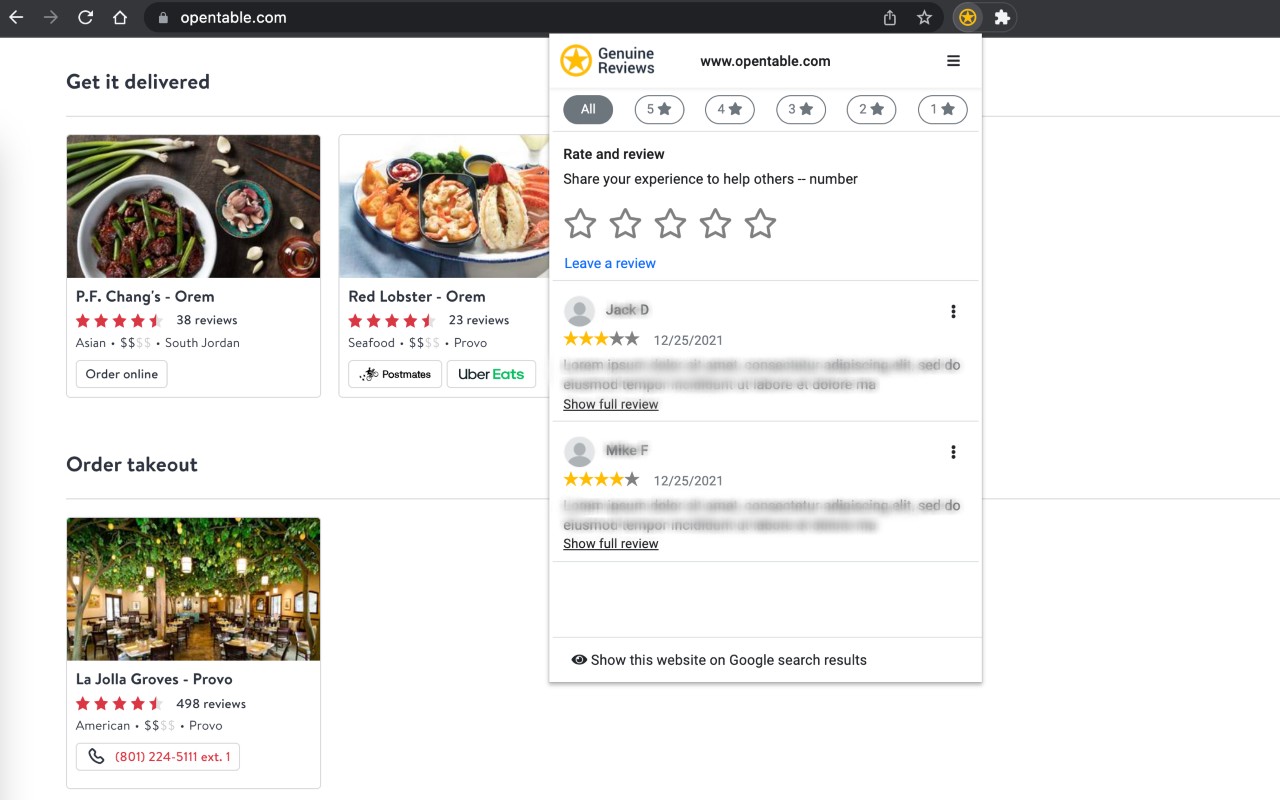This is a detailed screenshot of the OpenTable website visible on a computer screen, featuring the brand’s logo at the top and the address bar. Prominently, there is a "Get it delivered" banner.

At the center of the screenshot, a photograph showcases a bowl filled with a savory dish of brown-colored food garnished with fresh green vegetables on top, and accompanied by chopped vegetables behind it. Below the image, “P.F. Chang's Orem” is indicated, showing a star rating, with 38 reviews tagged to this Asian cuisine location in South Jordan. An "Order Online" button is readily available.

To the right, another enticing food image displays what appears to be a shrimp dish paired with a sauce and assorted vegetables. Captioned with “Red Lobster, Orem,” this entry highlights a star rating, alongside 23 reviews for this seafood restaurant located in Crow Hole. There are direct options for ordering via Postmates and Uber Eats prominently positioned below this image.

Continuing down the left side of the page, a call-to-action reading "Order takeout" draws attention. Adjacent to this, a photo of an empty restaurant space is provided featuring tables, chairs, overhead trees, leaves, and lamps, evoking a serene ambiance. The establishment is identified as “La Jolla Groves, Provo” with an impressive 498 reviews. This American cuisine restaurant is located in Provo, with a phone number, depicted by an adjacent phone icon, available for potential inquiries or reservations.

To the right side of the page, there is a section labeled "Genuine Reviews" by OpenTable.com, encouraging users to "Rate and Review" and share their experiences to assist others. This section includes functionality for users to leave a star review for businesses depicted on the page.

The overall layout of the screenshot integrates restaurant options with user review functionalities, facilitating both browsing and immediate action for viewers looking to order or evaluate dining experiences.